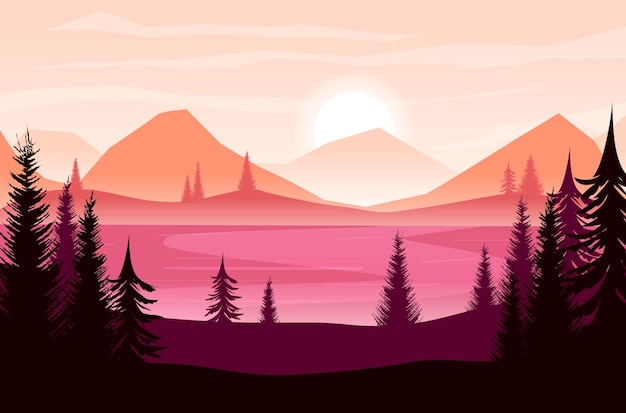This vibrant digital artwork depicts a vividly colored landscape at sunset. The scene showcases a forest surrounding a pink-colored lake, with distinct layers of trees and mountains. In the foreground, silhouetted black trees, likely birch, pine, or fir, stand out against the brilliant hues. Beyond these trees, a second layer of purple trees frames the water, which is rendered in shades of pink and salmon, highlighted in lighter pink. Distant hills, adorned with more trees, transition into a coral tone before reaching a striking orange mountain range. As the brilliant sun sets behind the peak of the mountains, it casts a radiant glow across an orange to pale-orange sky, complemented by creamy white clouds. The blend of black, purple, pink, salmon, coral, orange, and cream colors creates a vivid, almost surreal atmosphere, lending a distinctive animated quality to the scene.